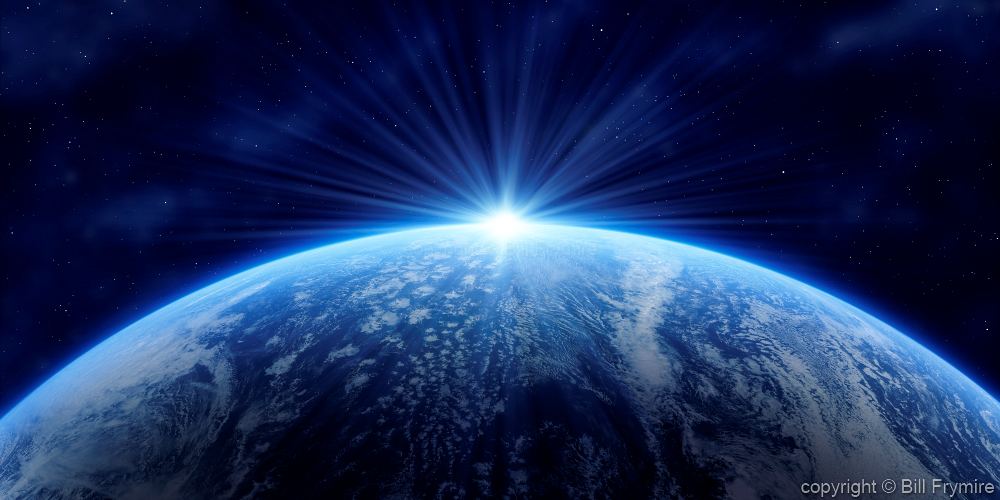The image is a detailed computerized rendering of a planet, reminiscent of Earth, viewed from space. Dominating the bottom half of the image, the planet's top third stretches from left to right, framed against a deep midnight blue background filled with countless white speckles, representing distant stars. The planet itself radiates with hues of blue and white, suggesting oceans and cloud cover, though no identifiable continents are visible, hinting it might be an imaginary world. At the center top of the horizon, there’s a brilliant light source, possibly a sun, emitting rays that disperse in all directions, creating a striking lens flare effect. Additionally, a blue nebula extends from the left side upwards to the top left and towards the center, with a separate nebula visible off to the right. The captivating visual is further accentuated by a copyright notice in the bottom right corner, crediting Bill Freymire.